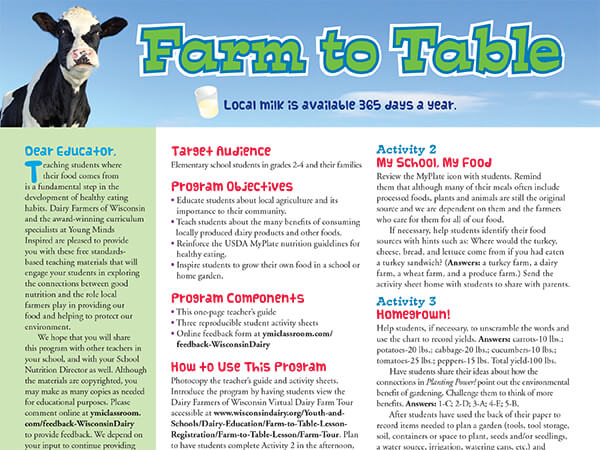The landscape image features a soothing sky-blue background with scattered clouds, stretching from the top left to the top right corners. Dominating the scene is a black and white cow gazing directly forward, positioned prominently on the left side. Above the cow, the text "Farm to Table" is displayed in vibrant green letters with a white outline. Beneath this text, an image of a glass of milk is accompanied by the caption "Local milk is available 365 days a year," emphasizing the year-round availability of locally-sourced milk. 

On the left side, a detailed letter addressed to educators is introduced with “Dear Educator” in blue. The letter underscores the importance of teaching students about the origins of their food to foster healthy eating habits. It mentions that the award-winning curriculum specialists at Young Minds Inspired have developed free standard-based teaching materials designed to engage students in understanding the role of local farmers in nutrition and environmental protection.

The middle and right sides of the image are divided into different sections with headings in red. These sections include "Target Audience," "Program Objectives," "Program Components," "How to Use this Program," and specific activities like "Activity 2: My School, My Food" and "Activity 3: Home Grown," each with additional explanatory paragraphs. Additionally, a chart offers guidance on effectively implementing the lesson plan, making it a comprehensive educational resource geared towards teaching children about the origin of milk and the vital role of farmers.